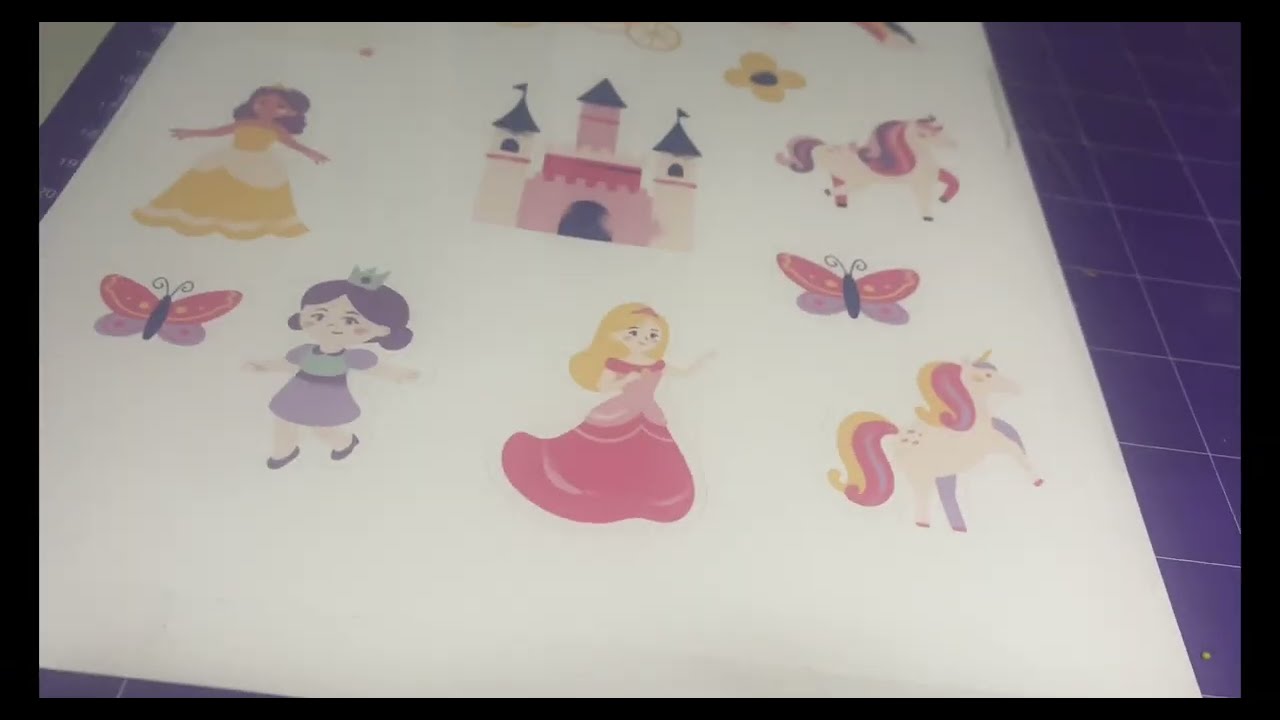The image depicts a large, unrolled sheet of white paper placed on a dark, blue-tinted cutting mat with white grid lines, giving it a professional feel. The paper is adorned with various detailed, cartoon-like illustrations of princesses, unicorns, butterflies, and flowers. The princesses are dressed in long, medieval or Renaissance-style gowns: one in yellow, one in red, and another in blue, with additional details suggesting blonde and dark-haired figures, one of whom wears a crown. In the center of the sheet, there is a stylized castle featuring three towers with pink gates and red walls. Around each character and element, there is ample white space, potentially allowing the images to be cut out into separate decals or illustrations. It's not entirely clear whether the images are printed or painted, but their vibrant, thematic design suggests a fairytale motif.